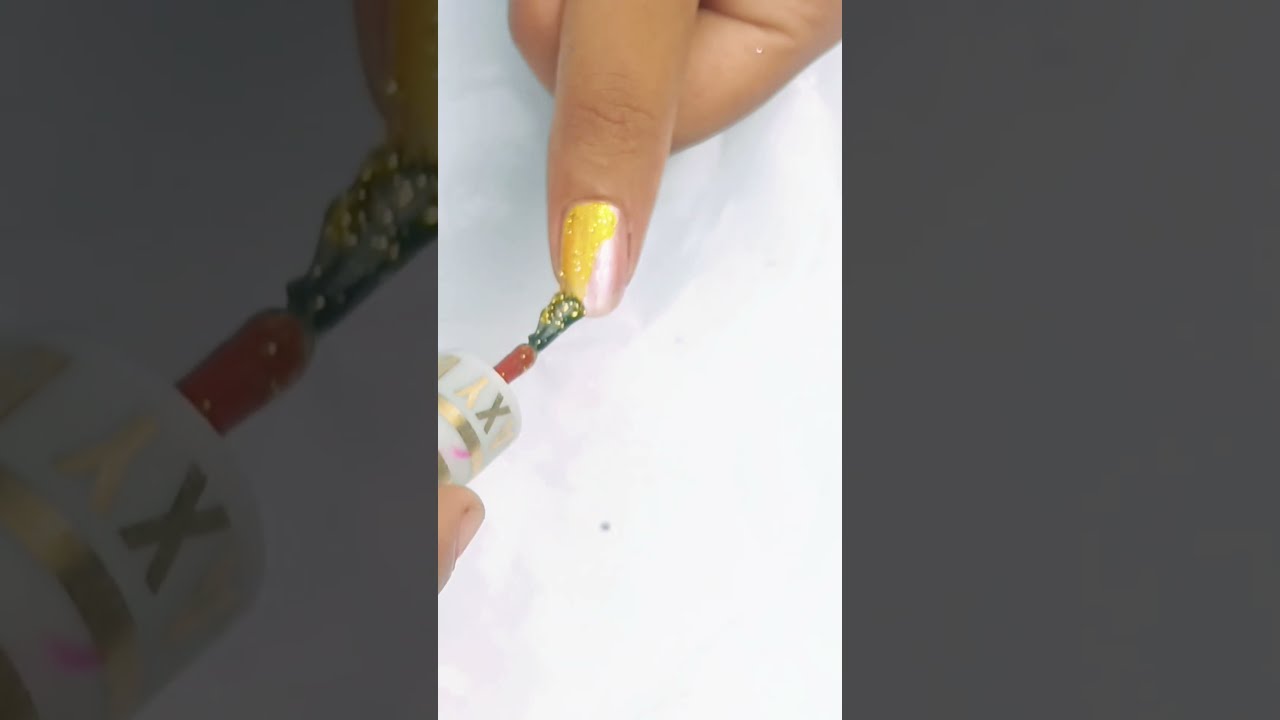The image captures a close-up shot, likely taken vertically for an Instagram or TikTok story, showing someone painting their thumb nail. The background is predominantly white, possibly a table or countertop, while the sides of the image appear gray and darker, adding contrast. The person's thumb protrudes from a clenched fist, extending into the frame from the top. The thumb already has a pink base layer, onto which the person is applying a glittery gold nail polish. A black brush with gold glitter on it, connected to a white bottle with gold lettering reading "Max," is being used to apply the polish. The scene is well-illuminated, casting the thumb's shadow onto the white surface, emphasizing the meticulous nail-painting process.